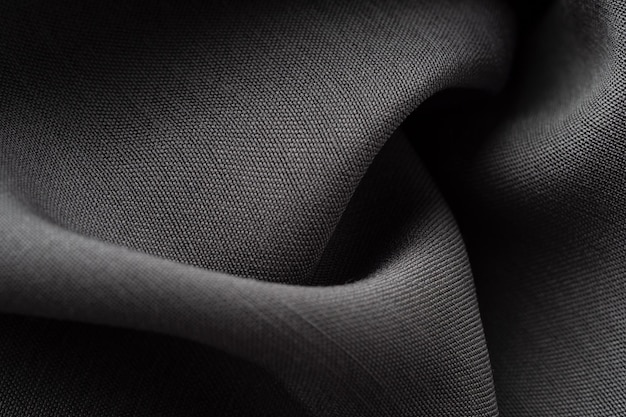This photograph showcases a medium soft gray fabric, exhibiting a tight weave, potentially suggesting a polyester material or a pair of slacks. The fabric appears bunched together with three distinct folds, giving it a slightly relaxed texture. The light source softly illuminates parts of the fabric, creating light shadows and subtle highlights, while a deep shadow envelops the bottom left-hand corner, resulting in total blackness. The material, seemingly thick and possibly burlap-like, portrays a simplistic composition without any words, artist trademarks, or watermarks. Vertically and horizontally aligned stitching, characterized by intermingled dark and gray dots, forms a distinctive pattern across the fabric. Shadows interplay with the folds, creating darker regions, notably in the left, top, and right corners, and collectively forming a shadow resembling the letter T.